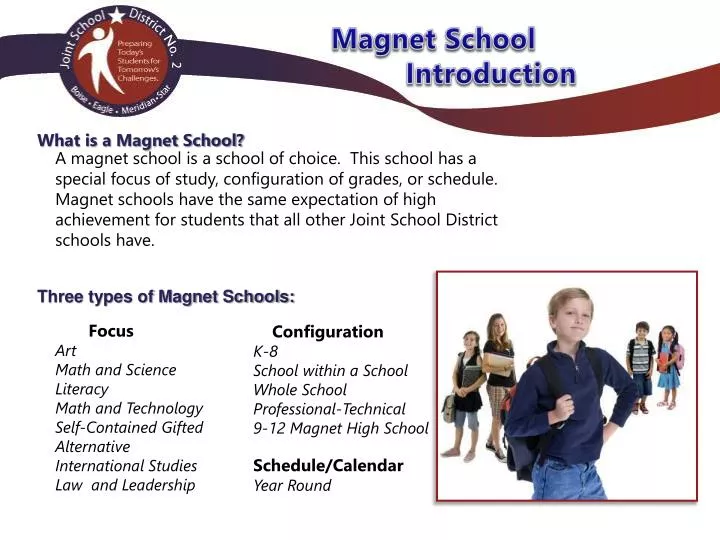The infographic titled "Magnet School Introduction" features a prominent blue text header at the top, accompanied by a black and red banner with a circle on the left side indicating "Joint School District Number 2." Below the main title, a comprehensive description outlines what a magnet school is—highlighting that it's a school of choice with a special focus on study areas, grade configurations, or schedules. The infographic emphasizes the high achievement expectations for students within the magnet school system.

Key sections of the infographic include detailed descriptions of the "Three Types of Magnet Schools"—Focus, Configuration, and Schedule Calendar—each presented with accompanying text and visual elements. A visual motif of a blue ribbon transitioning to red is present at the top, adding a vibrant touch.

In the lower right-hand corner, there's a picture of several students. Prominently featured is a blonde child in a blue sweatshirt and jeans, posing confidently with a backpack. Surrounding this child are four other students, each holding books and papers, showcasing a typical school scene.

Additionally, the infographic includes a logo in the upper left, with the school district's motto "Preparing Today's Students for Tomorrow's Challenges" displayed within a red circle, accompanied by a white figure. The overall layout is designed to inform and attract parents and prospective students by explaining the unique benefits and configurations of magnet schools. The background is white, allowing the mixed colors of the text and visuals—mostly blues and reds—to stand out clearly.